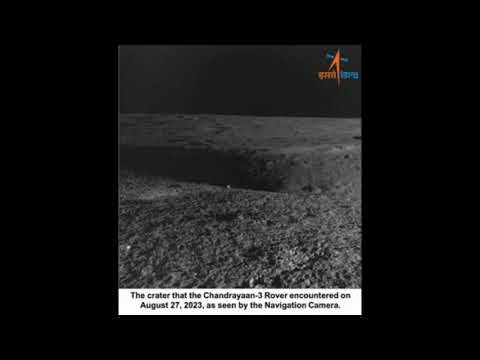The image depicts a dark, monochromatic photograph resembling the moon’s surface, characterized by a rocky, gray, and sandy terrain with a notable crater at its center. The photograph is framed by a thick black border that is heavier on the right and left edges, and thinner at the top and bottom, emphasizing the central lunar-like landscape. The upper right-hand corner features a blurry, sideways red check mark along with an indistinct logo in red and blue, possibly in a foreign language. The top of the image is particularly dark, suggesting a vast, black backdrop consistent with a space setting. At the bottom of the image, within a white strip, a caption in black text reads, "The crater that the Chandrayaan-3 rover encountered on August 27, 2023, as seen by the navigation camera."